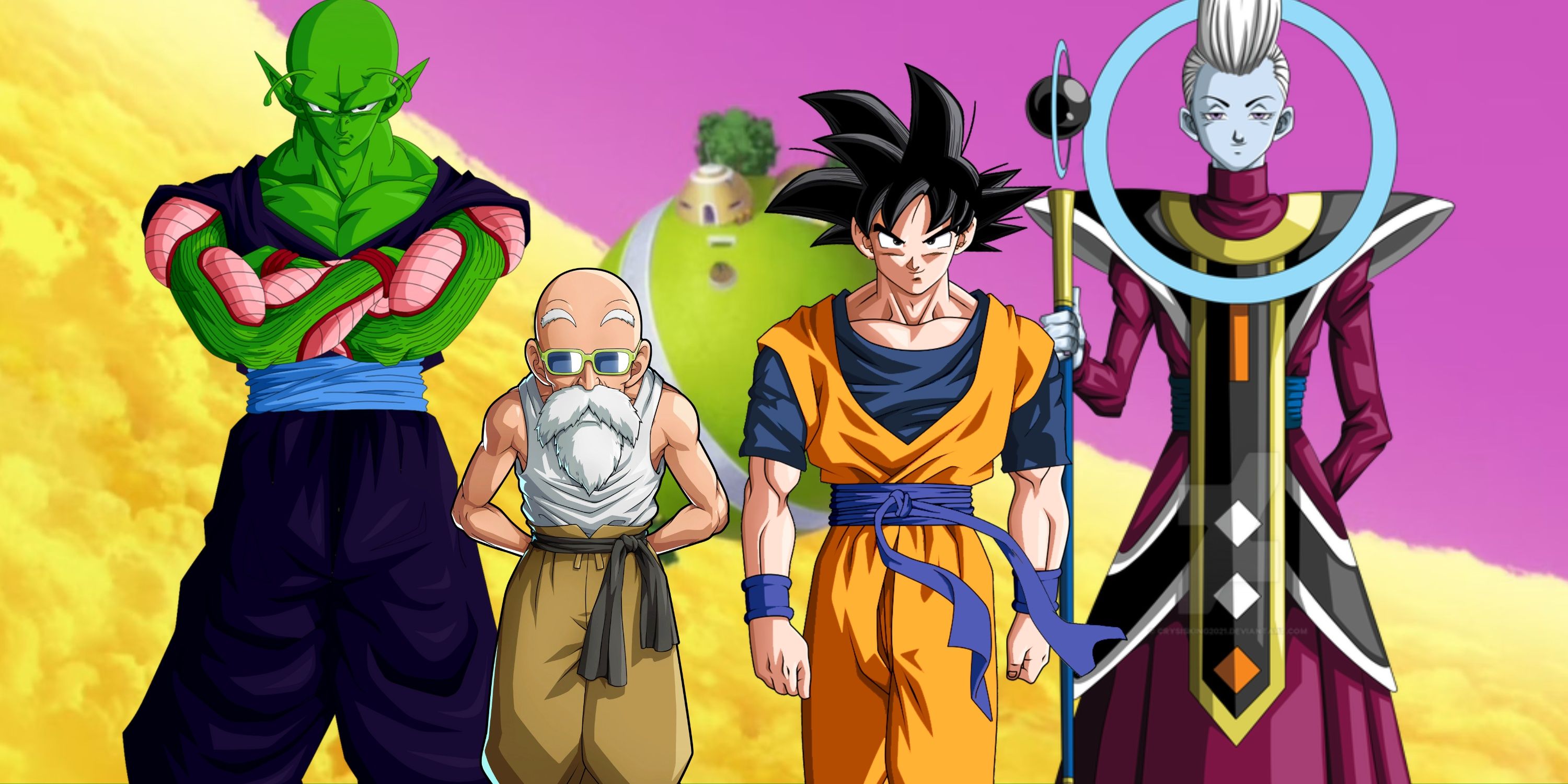A digitally-created collage features characters from the Dragon Ball Z series set against a surreal background. Central in the foreground stands Goku, the primary protagonist, recognizable by his spiky black hair, blue shirt, and orange jumpsuit with a purple belt. To his left is an elderly man sporting a white tank top, beige pants, sunglasses, and a bushy white beard and mustache, his hands clasped behind his back. Further to the left stands a muscular, green-skinned figure reminiscent of Piccolo, characterized by his bald head, pointy ears, and mixed black and pink arm and chest details, wearing purple pants with a blue waistband. On Goku's right is a unique character with blue skin, white hair, black shoulder pads, and a purplish-pink dress, holding a staff with a black orb at its end. The background boasts a vibrant array of colors with yellow cloud formations against a pink-purple sky. In the backdrop, there is a round green planet-like structure, adorned with a small house, tree, and an object resembling a dog's dish. The collage appears meticulously crafted, likely through Photoshop, combining individual character images into a cohesive group scene.